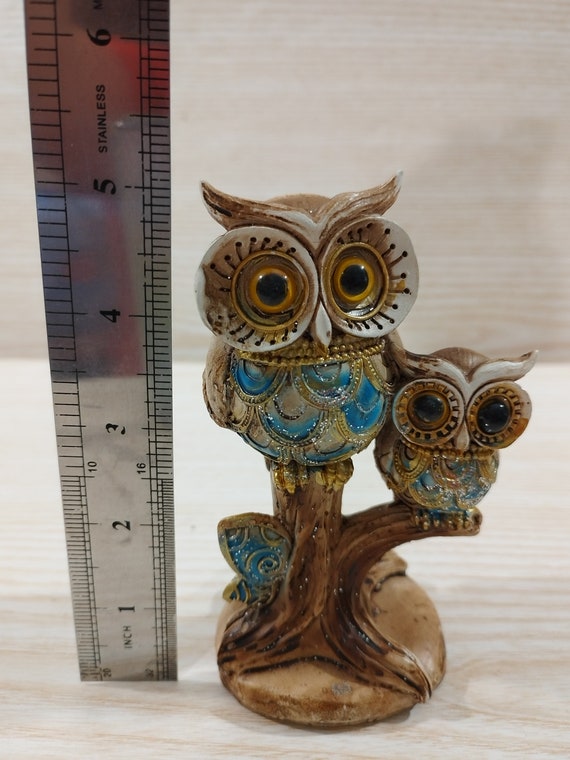The image showcases a detailed, close-up photograph of a decorative statue featuring two intricately designed owls perched on a tree stump. The larger owl, distinguished by its enormous golden eyes and expressive, thick eyebrows, sits higher on the stump, while a smaller owl with equally striking features perches lower down the branch. Both owls display a vibrant mix of blue and gold on their feathers. A delicate blue butterfly can also be seen on the side of the tree branch. The entire sculpture, resting on a stone-like round base, is positioned beside a vertically placed silver ruler, clearly showing its height as exactly 5 inches. The background of the image is an off-white color, highlighting the artistic and abstract design of the ceramic or pottery piece.